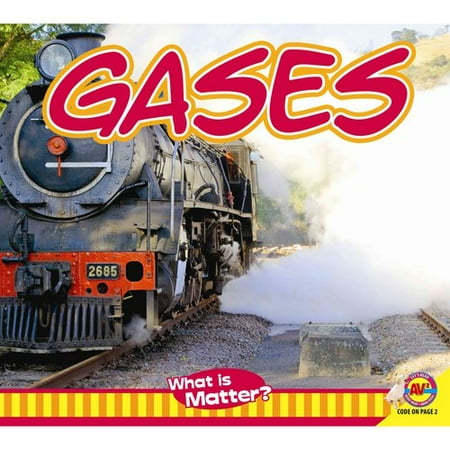This educational poster features a black coal-powered train locomotive prominently positioned on the left side, emitting billowing steam or smoke. The front of the locomotive showcases a red cow catcher with the numbers 2685 on a small plaque, and a significant light near the top. At the very top of the image, large red lettering with a yellow outline spells out "GASES." The background includes a touch of nature with a few trees visible in the upper left-hand corner. The bottom of the poster is bordered in orange and yellow, with an oval-shaped red section containing white text that reads, "What is MATTER?" In the bottom right corner, a small logo featuring a bird and the text "AV CODE on page 2" hints at its educational purpose.